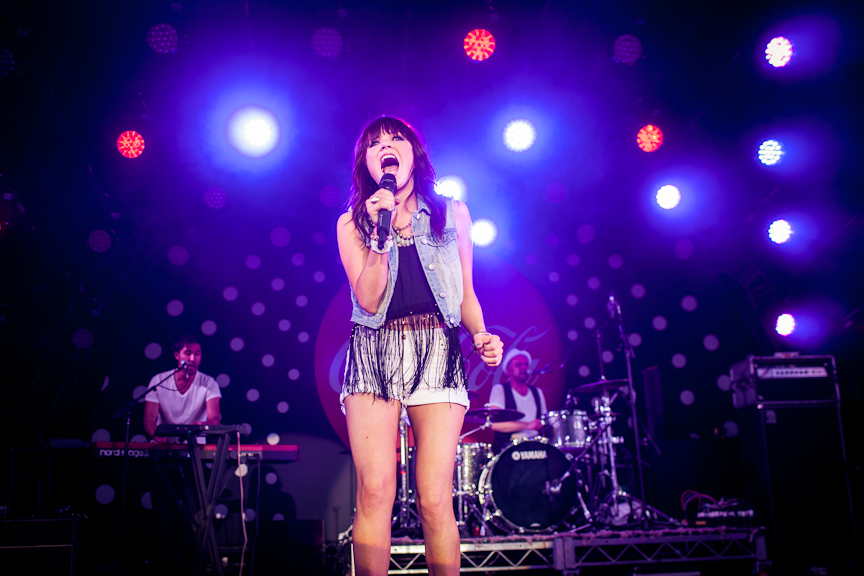A young female singer stands energetically on stage, her mouth wide open, passionately singing into a black microphone. She is dressed in a striking combination of a denim vest over a black shirt, black tassels adorning it, paired with high-waisted white shorts secured with a leather belt. Hulking behind her is a drummer, seated at a black Yamaha drum kit. The drummer sports a white hat, a white shirt, and a black vest. To the left, a young man with black hair operates a keyboard positioned on a stand. A large bass amplifier cabinet, most likely an 8x10, is situated to the right side of the stage. Dominating the backdrop is a prominent red Coca-Cola logo with white text, adding a burst of bold color to the scene. Surrounding the performers are a series of spotlights, casting dynamic beams of light on the stage. The overall setting appears to be a lively concert, brimming with elements in hues of red, white, black, brown, and silver, contributing to the vibrant atmosphere.